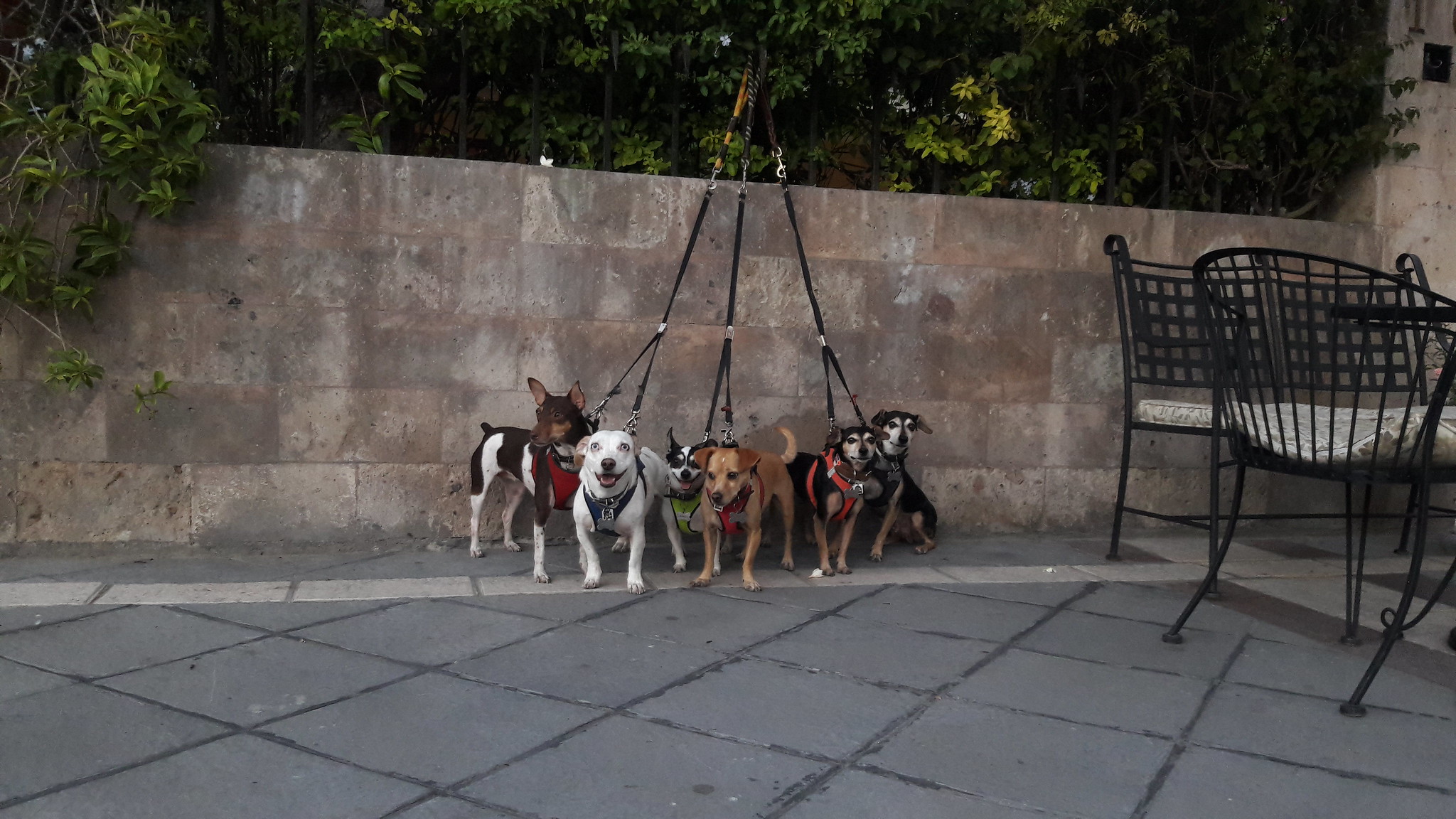The photograph captures an outdoor scene featuring six leashed dogs of various breeds and colors, all arranged in front of a large concrete wall composed of rectangular squares. Behind the wall, a dense area of green trees is visible, with several branches extending over the wall. The dogs' leashes are attached to these branches, ensuring they remain stationary on the patio, which has a checkerboard pattern of cement tiles.

From left to right, the first dog is a Jack Russell type with a brown head and a black and white body. Next is a small white dog with distinctive black and brown ears, followed by another tiny black and white dog with a predominantly white body. The fourth dog is entirely brown, standing out in the group. The two dogs furthest to the right are nearly identical, both having black bodies with light brown legs and white heads. While most of the dogs are standing, the last dog on the right is seated. All dogs are looking attentively towards the camera.

The right side of the image includes patio furniture, specifically black wrought iron chairs with white patterned cushions, adding to the outdoor setting. The overall scene suggests a moment of calm as these small, diverse dogs await their next adventure.